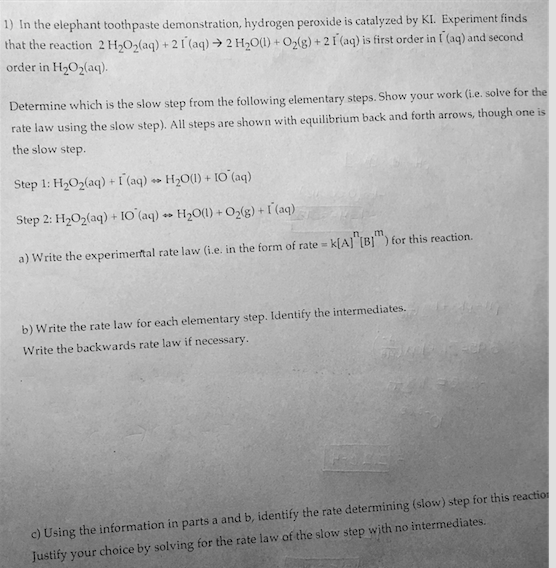This image portrays a printed worksheet, likely from a science class, featuring a detailed chemistry problem. The paper is standard white with typed black text and begins with a clear "1)" indicating the first question. The assignment elaborates on the "elephant toothpaste demonstration," explaining that hydrogen peroxide is catalyzed by K1. The problem includes chemical equations, particularly noting that 2H2O2(aq) reacts, implying complexities in its orders of reaction—first order in one of the reactants and second order in H2O2(aq). The worksheet instructs students to determine the slowest step among given elementary steps and to show their work in solving for the rate law using the identified slow step. Additional sub-instructions are labeled A, B, and C. On the reverse side, slight bleed-through marks from handwritten notes or pencil imprints are noticeable, reinforcing that this is likely a homework assignment needing completion.